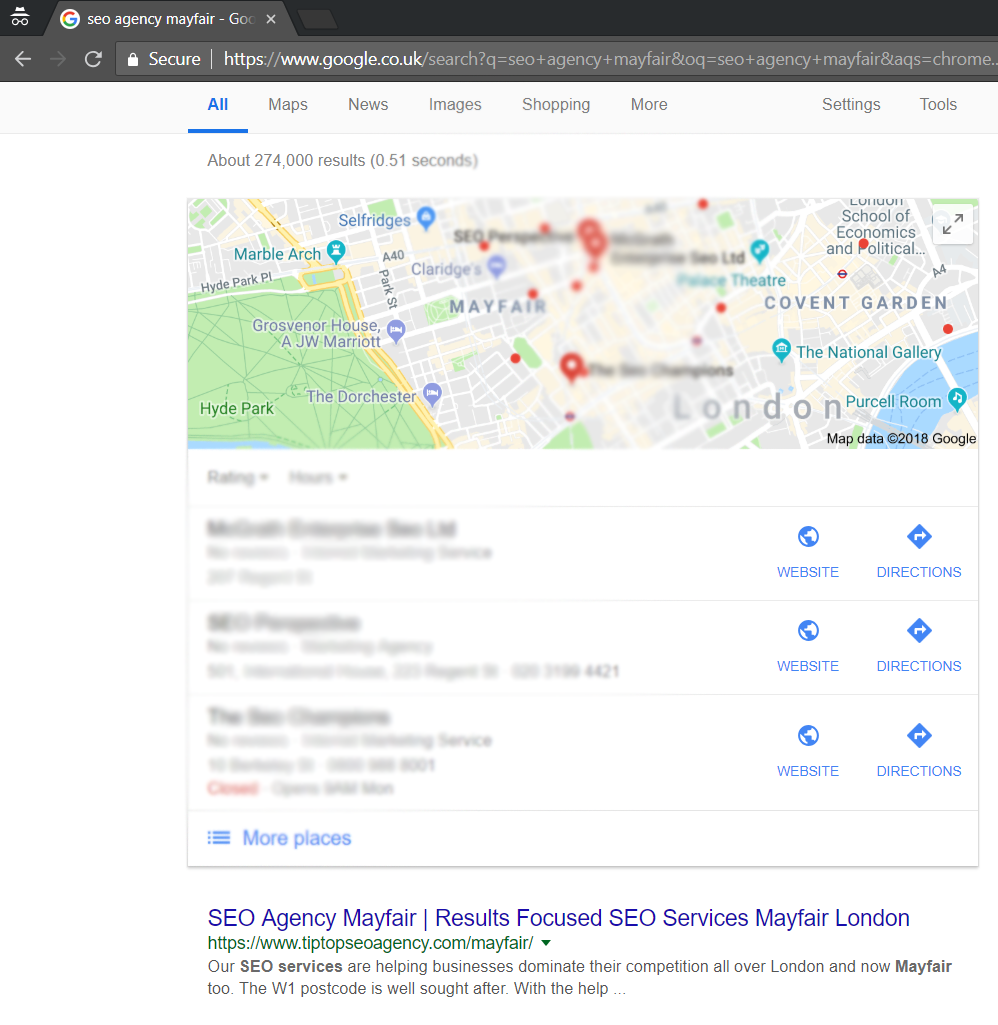The image is a screenshot of someone using Google Maps on a computer in incognito mode. The incognito mode is evident from the distinctive icon in the upper left-hand corner, featuring a hat and glasses on a black background. This choice of browsing mode suggests the user is attempting to maintain some level of privacy.

The browser displays an active tab titled "Agency Mayfair," with the standard navigational tools such as the back button, refresh button, and the address bar, which includes a gray "Secure" label indicating a secure connection.

In the main section of the screenshot, Google Maps is open, showing a map of London. The map includes notable landmarks such as Hyde Park on the left. Most of the interface details are blurred out, including specific locations and search results, to further anonymize the content.

Beneath the map, some search results are partially visible. On the right-hand side of these results are buttons including “Website,” indicated by blue text, and a white directional arrow icon surrounded by blue with the word "Directions" underneath in red and blue. The page indicates about 247,000 results in 0.15 seconds, demonstrating the efficiency of the search.

Overall, this detailed screenshot reveals various layers of Google's user interface while hinting at the user's intent to maintain privacy through incognito mode.